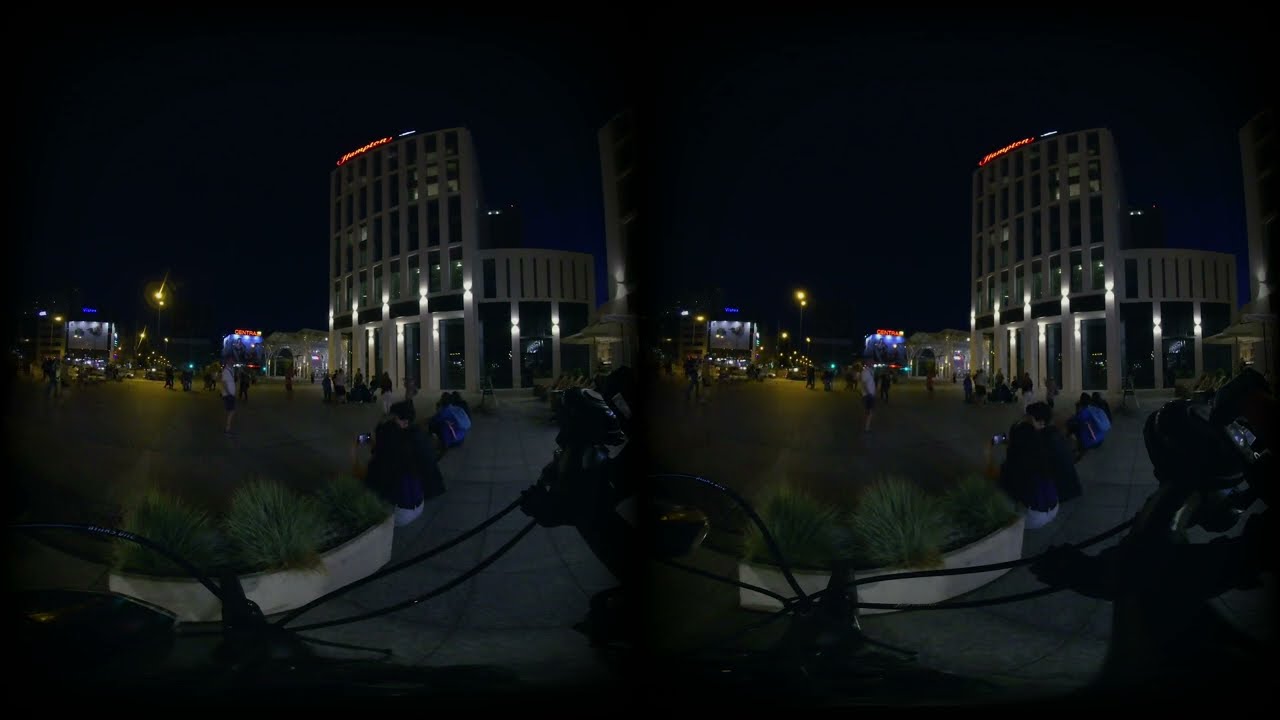This image depicts a nighttime city square, shown in two side-by-side, curved photographs separated by a black line. The square is paved with gray, square-shaped tiles and features a central planter containing three green plants. The scene is bustling with activity; numerous people are seen walking, standing, sitting, and using their phones. In the backdrop, a skyline of varying building heights is visible, some adorned with illuminated signs and colorful lights, including blue and red hues. One prominent building features distinguishable orange light strips near its roofline. Streetlights cast a warm yellow glow, enhancing the lively yet serene atmosphere of the evening cityscape.